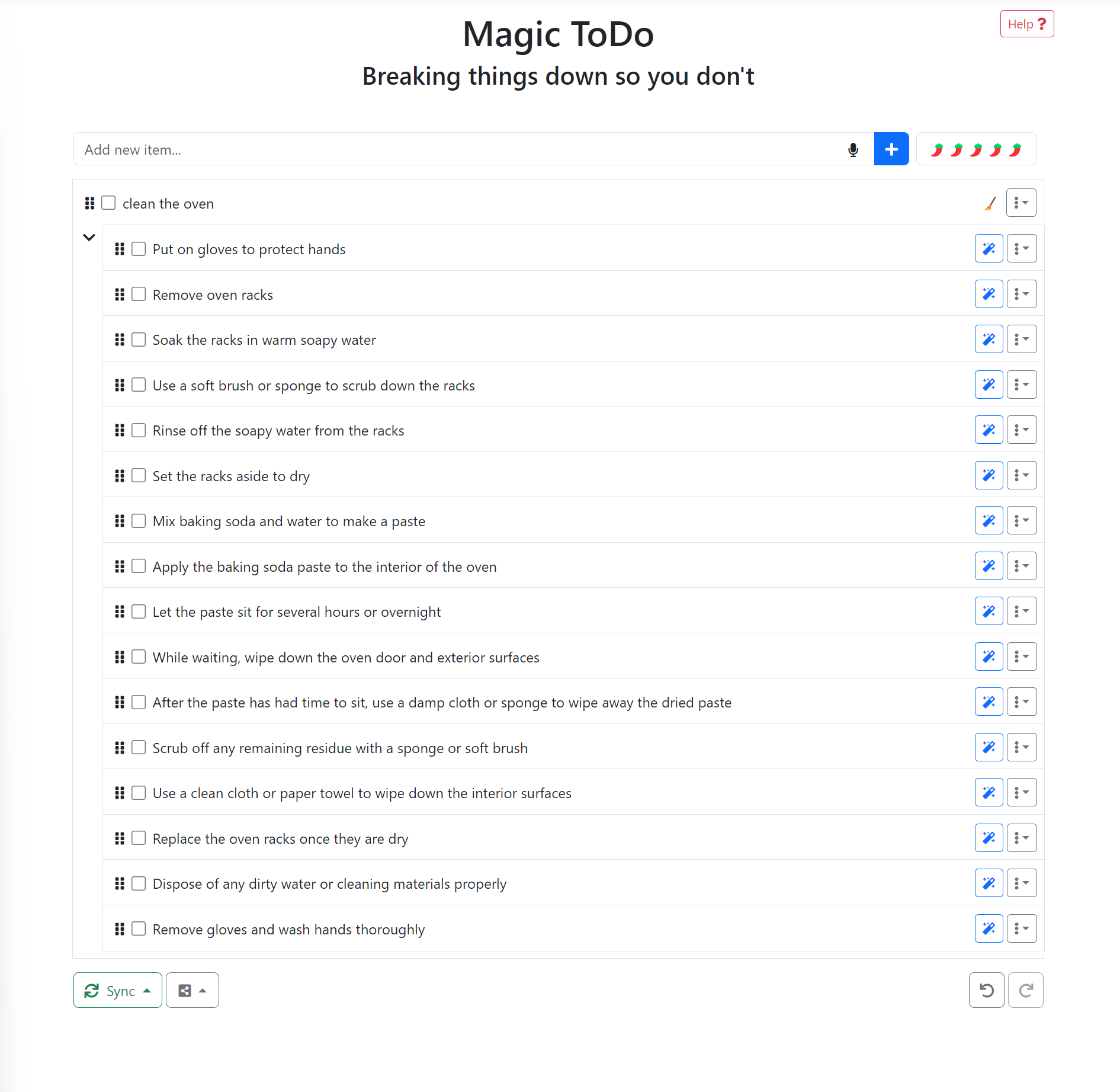This image is a detailed screenshot captured from a computer or tablet device, displaying an open window within an application. The interface features a white background with a table-style format and an organized grid layout. The title at the top reads "Magic To Do: Breaking Things Down So You Don't Have To," highlighting the application's purpose of simplifying task management. Positioned at the top right corner is a prominent red "Help" button, offering assistance to users.

The central part of the screenshot consists of a structured list, resembling a to-do list, with functionality for adding new items at the top. Each task on the list is accompanied by descriptive text explaining the necessary steps, and adjacent to these descriptions are controls for managing each item. On the right side of each entry, users can either erase the task or click on a button with three vertical grey dots, revealing a dropdown menu with additional options.

The specific to-do list displayed focuses on the detailed steps required to clean an oven. It includes instructions such as "Put gloves on hands to protect hands," "Remove the oven racks," "Wash the oven racks," among others. The sequence continues through all the necessary actions until the final step, which is to replace the oven racks once they are dry.